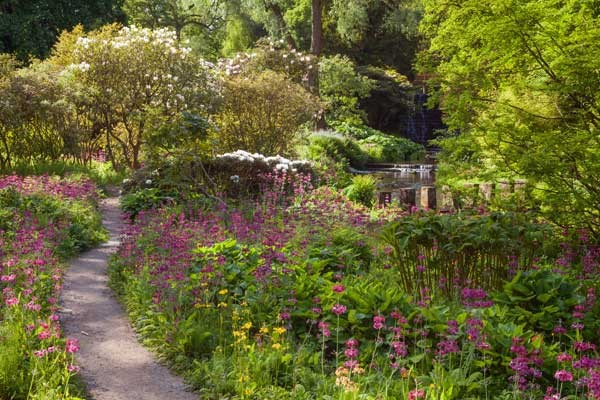In this photograph, we're looking at a serene and picturesque park, likely captured during spring or summer. On the left-hand side, there is a curved winding path, initially bending to the left and then to the right before straightening out. This pathway is surrounded by tall, vibrant flowers, predominantly purple in color, resembling wild lavender, and interspersed with lush green shrubbery. Additionally, some pink flowers can be spotted among the greenery.

In the background, several trees can be seen, their branches adorned with varying shades of green leaves, ranging from light to dark hues. One prominent tree features delicate white blossoms on its upper branches, possibly indicating a fruit tree in bloom. Beyond the trees, an intricate building structure with about seven or eight windows or doors is visible, adding a touch of architectural charm to the natural landscape.

To the right of the scene, there is a small pond accompanied by an artificial waterfall, contributing to the tranquil atmosphere of the park. The water cascades gently down, creating a peaceful ambiance. This idyllic setting, with its combination of vibrant floral displays, lush greenery, and calm water features, evokes the essence of a classic English country garden.